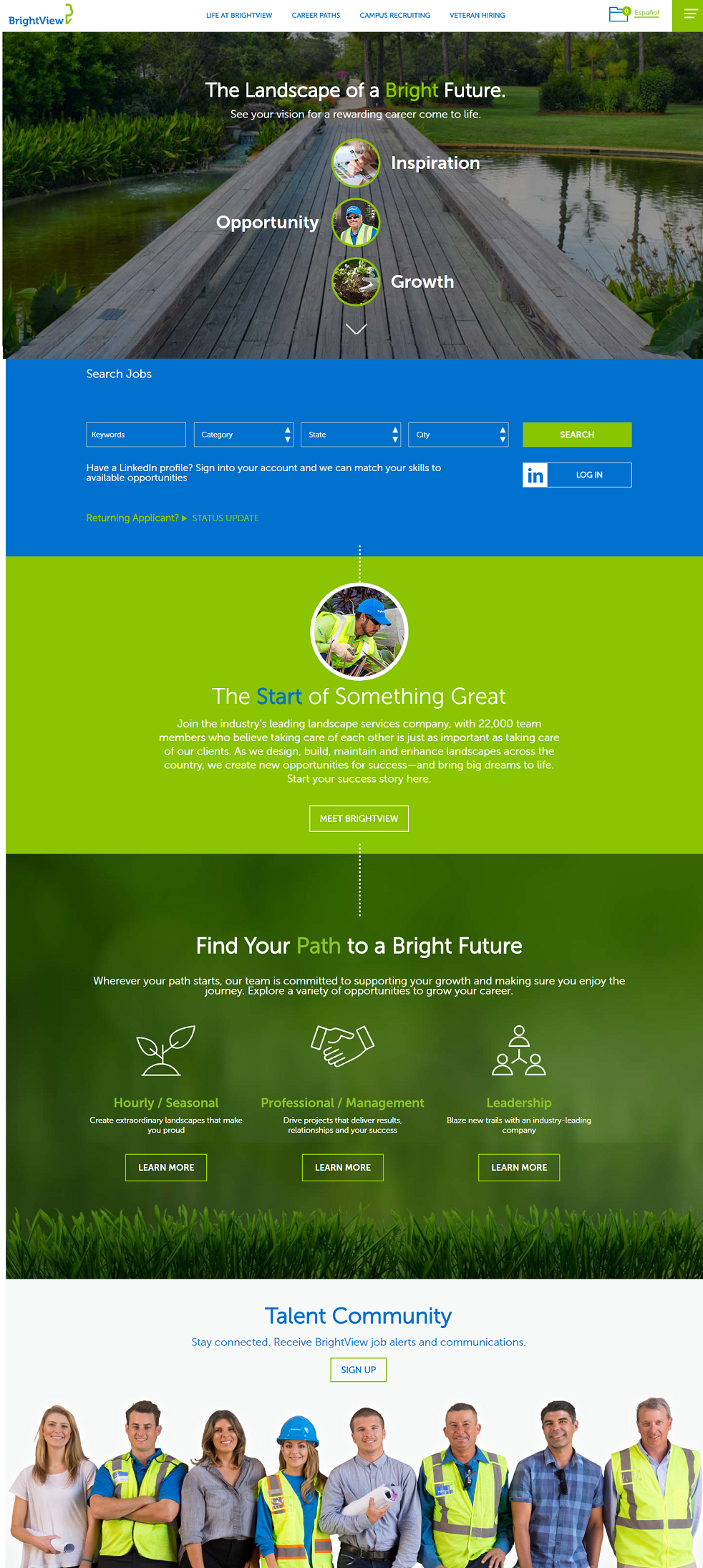The image depicts a webpage with the heading "Brightview" positioned at the top left corner. Directly to the right, there are four navigation tabs labeled as follows, from left to right: "Life at Brightview," "Career Paths," "Campus Recruiting," and "Veteran Hiring." Below these tabs, a prominent heading reads, "The Landscape of a Bright Future," accompanied by the subheader, "See your vision for a rewarding career come to life."

Beneath this text, three circular images are displayed in a vertically stacked arrangement. The topmost circle, labeled "Inspiration," features a close-up shot of a hand writing. The middle circle is labeled "Opportunity" and shows a man wearing a blue hat. The bottom circle, titled "Growth," contains an image of a plant sprouting from soil.

Further down the page, there is a section titled "Search Jobs." This section includes four search tabs, followed by a button labeled "Search."